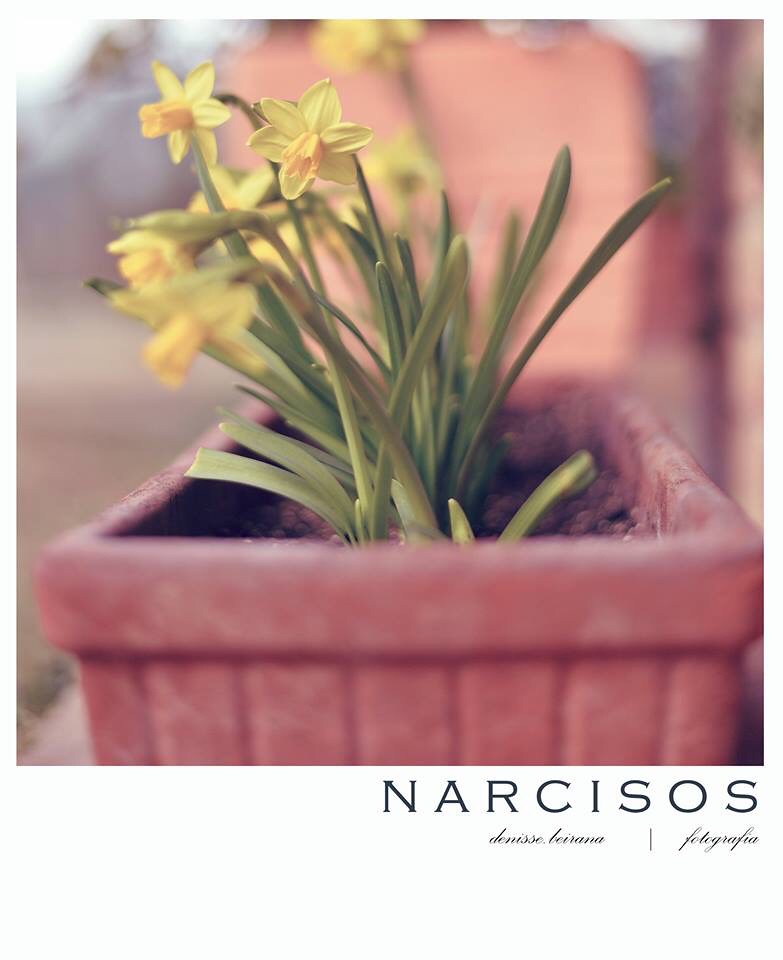The image depicts a terracotta planter, rectangular in shape with vertical ridges along its sides and a beveled lip encircling the top. Planted within the pinkish-clay colored pot are vibrant yellow daffodils, some with orange centers. The flowers have long green stems, several inches tall, with most topped by yellow blossoms, though a few stems remain bare. The planter is positioned such that we view it from the narrow edge, with the wider side receding into the background. The soil inside is visible, reinforcing the natural planting. In the bottom right-hand corner of the image, in black lettering, the word “Narcissus” is visible, followed by the name “Denise Beirana” and “Fotografia.” The backdrop features a blurred mix of white and blue sky, with hints of green grass to the left and possibly a building or shed directly behind, suggesting the setting is outdoors.